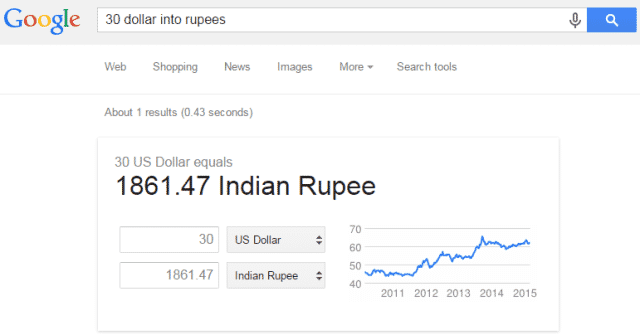The image depicts the Google search interface featuring the iconic multicolored Google logo against a gray rectangular background. The logo displays the blue 'G', red 'O', yellow 'O', blue 'G', green 'L', and red 'E'. Beneath the logo is the search box containing the query "$30 into rupees." To the right of the search box are a grayish-black microphone icon and a blue rectangle with a white search magnifying glass within it.

Below the search box are navigation options including "Web," "Shopping," "News," "Images," "More" with a dropdown, and "Search tools." Further down, a faint gray line separates these options from the search results. The result reads "About 1 result (0.43 seconds)," with the seconds in parentheses. The conversion result shows "30 US dollars equals 1861.47 Indian rupees," displayed with "30" in a text box and "1861.47" in another text box below it. Next to this conversion, there are up and down arrows for selecting different currencies in both fields to compare various exchange rates.

To the right, a chart visualizes the currency exchange rates over time, with the years 2011 through 2015 marked along the x-axis and the values 40, 50, 60, 70 along the y-axis. The chart indicates that the exchange rate peaked around the end of 2013 to the beginning of 2014.